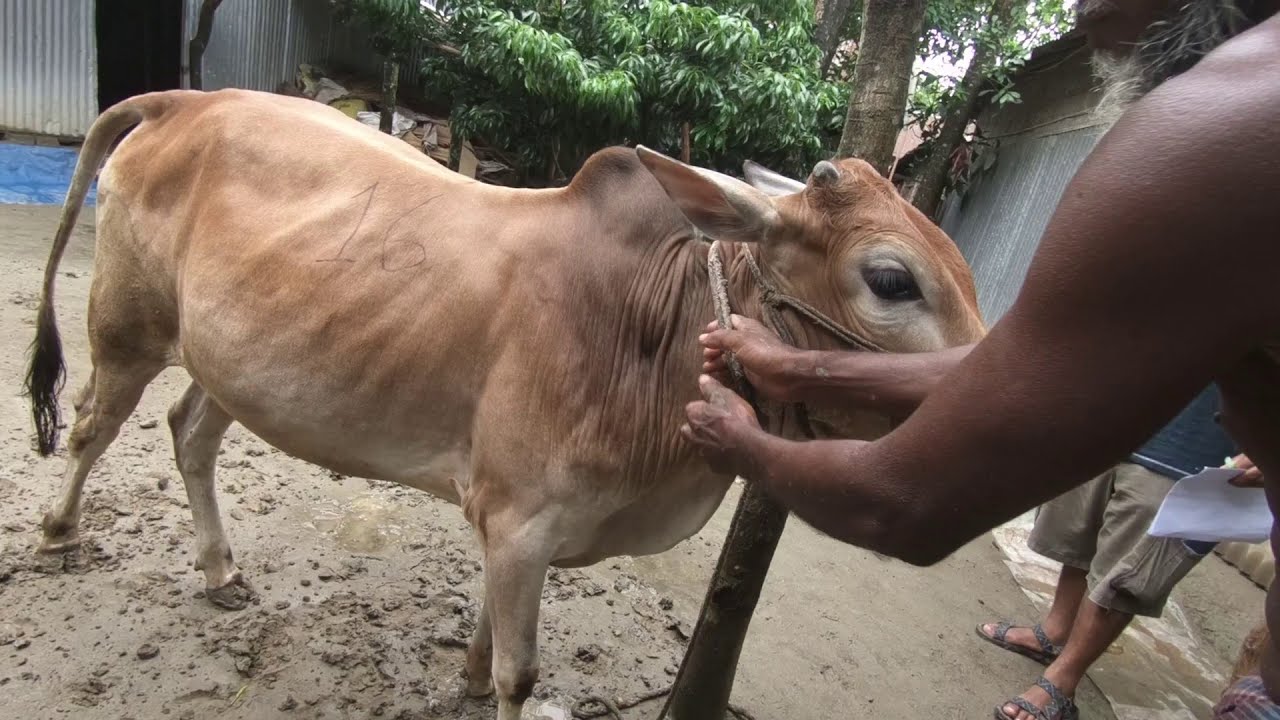In the photograph, a small cow, possibly a calf, stands facing to the right in an outdoor setting. The cow has a predominantly brown coat with some white patches and the number "16" is written on its side. The cow's ribs are somewhat visible, indicating that it may be a young or undernourished animal. A rope is tied around the cow's head, held by a dark-skinned person whose arms and shoulders protrude into the frame. Another person's legs are visible next to the cow's handler. The ground is gray and muddy with patches of dug-out soil. In the background, there are thin building structures and some green-leaved trees.